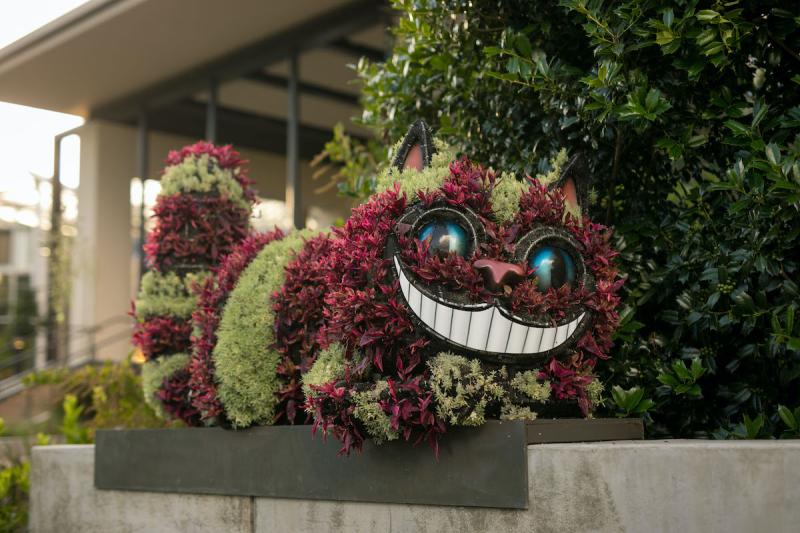The image depicts a detailed outdoor scene in front of a building with a concrete planter. The planter, made of cement, features an intricate arrangement of plants. On the right side, a mix of vibrant green and darker green plants is visible, while the middle section showcases lighter green plants interspersed with red plants. The planter has been fashioned into the striking figure of the Cheshire Cat, complete with accessories that create big blue eyes, a black-outlined large mouth with white teeth, a nose, ears, and a tail, mimicking the famous feline's striped pattern using alternating red and green plants. This imaginative creation, held together likely by a metal frame, stands out vividly against the backdrop of the white building, which includes metal railings and a green gauge. This lush and creative display not only enhances the aesthetic of the building's exterior but also adds a whimsical touch for passersby to enjoy.